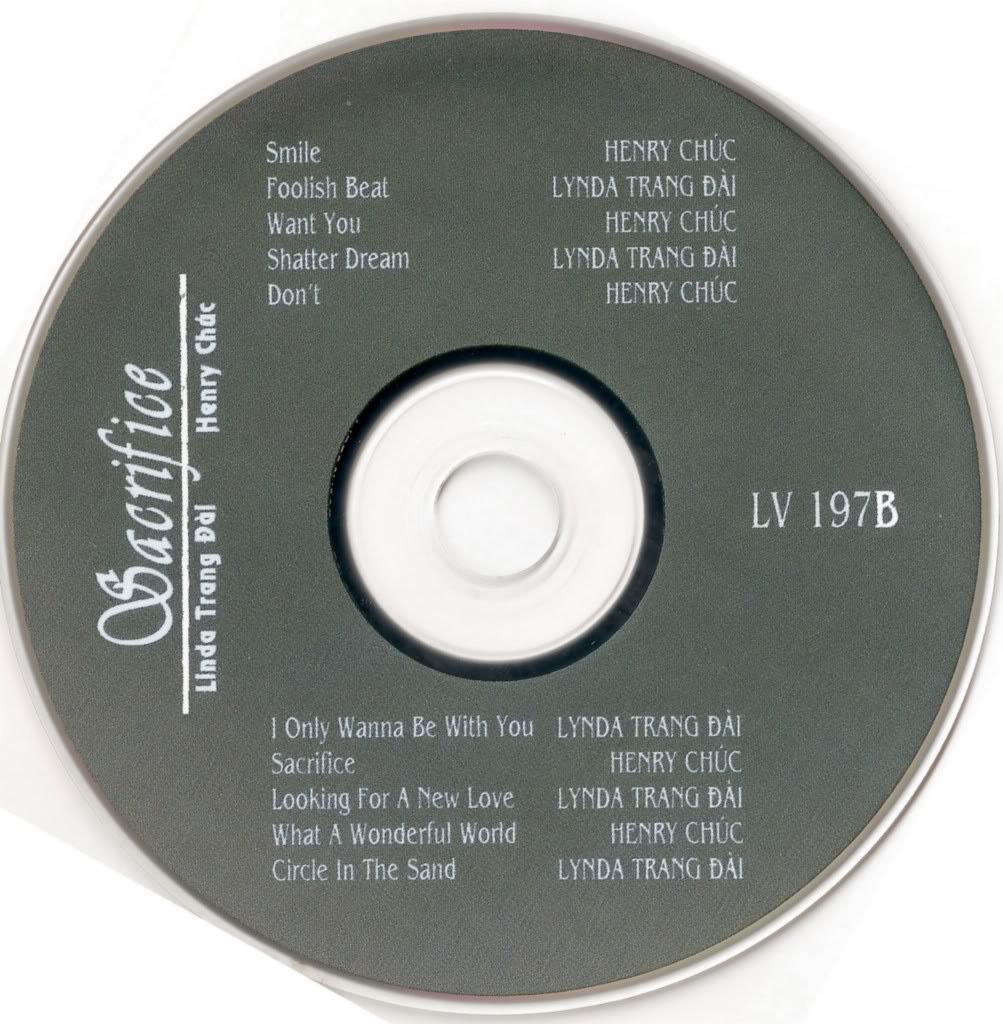This image features the front view of a black audio CD with white text. In the middle right section, the code "LV197B" is clearly printed. The album is titled "Sacrifice" and features performances by Linda Trang Dai and Henry Chuck. Near the left margin, written vertically, are the words "Sacrifice" followed by a line, then Linda Trang Dai and Henry Chuck.

The track list is detailed on the CD, starting at the top with "Smile" by Henry Chuck, followed by "Foolish Beat" by Linda Trang Dai, "Want You" by Henry Chuck, "Shattered Dream" by Linda Trang Dai, and "Don't" by Henry Chuck. Continuing, the tracks include "I Only Want to Be with You" by Linda Trang Dai, "Sacrifice" by Henry Chuck, "Looking for a New Love" by Linda Trang Dai, "What a Wonderful World" by Henry Chuck, and "Circle in the Sand" by Linda Trang Dai.

The meticulous design and layout indicate that this is a musical CD album featuring collaborative works from both artists, with each track distinctly attributed to either Henry Chuck or Linda Trang Dai.